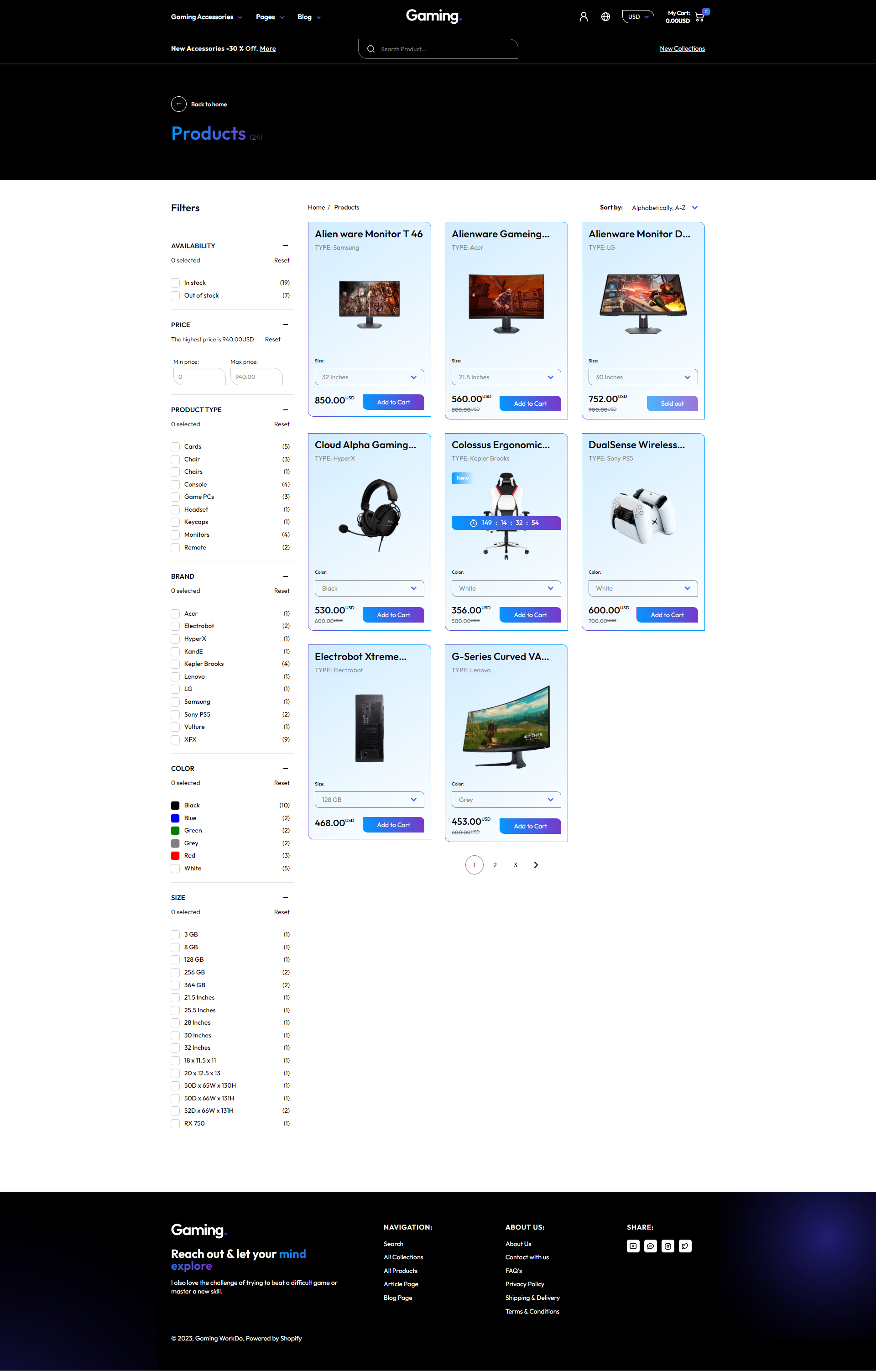This image is a screenshot from a website dedicated to gaming. The design features prominent black banners at both the top and bottom of the page.

At the top banner, the word "Gaming" is prominently displayed. To the right, there are several navigational dropdown menus labeled "Gaming Accessories," "Pages," and "Blog." The banner also highlights a special promotion: "New Accessories, 30% Off, More." A multicolored text link, transitioning from blue to purple, reads "Back to Home Products." Adjacent to this is a search bar with the placeholder text "Search product." Additionally, there are icons indicating a globe, a user profile, and a currency dropdown labeled "USD." A shopping cart icon displays "My Cart, 0," and the phrase "New Collections" is present.

To the left, a vertical sidebar menu provides various filters for refining the product search. These filters include availability options ("In Stock" and "Out of Stock"), a price range slider labeled "Maximum Price" and "Minimum Price," and product type categories such as "Cards," "Chairs," "Console," "Game," "PCs," "Headset," "Keycaps," and "Monitors." There are also options to filter by brand, color, and size.

The main content area of the screenshot shows the breadcrumb navigation "Home > Products," followed by an array of product panels organized in rows: three panels in the first row, three in the second row, and two in the third row.

At the bottom banner, once again labeled "Gaming," is the slogan, "Reach out and let your mind explore." Additional links for "Navigation," "About Us," and "Share" are provided, along with social media icons for easy sharing.

This detailed layout offers a comprehensive overview of the website's interface, showcasing its user-friendly design and extensive filtering options to enhance the shopping experience.